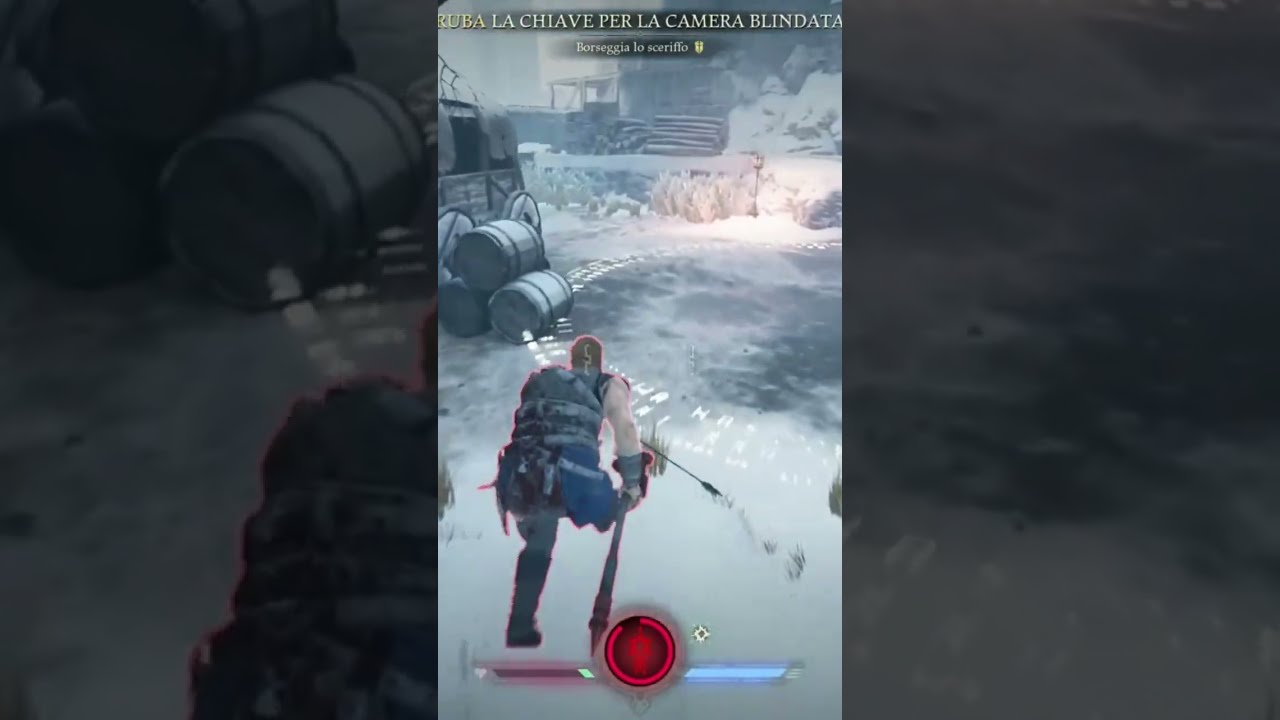The image is a horizontal rectangle featuring a video game scene divided into three vertically aligned parts: a left, right, and center panel. The left and right panels are dark, blurry, and appear to be zoomed-in portions of the center image, showing indistinct ground and rocks. The center panel is brightly lit and features a vertical rectangle with a clear depiction of a computer game. At the top of this middle panel, text reads "Ruba la Kieva per la camera blindata." Below this, there is a snowy scene with barrels on their sides and a wooden wagon with white wheels in the left foreground. In front of the wagon, a computer-generated character stands with his back to the viewer, holding a long weapon, possibly a sword or axe. He appears to be wearing blue and gray leather armor with numerous straps and metal wrist guards. In the bottom section of the middle panel, there is video game interface elements: a red circle, a red bar, and a blue bar, possibly indicating health or other game metrics. The background of the scene features a log cabin, stacks of timber, and rugged rocky terrain. Overall, the image combines a detailed game scene in the center with darker, less clear extensions of this scene on the sides.